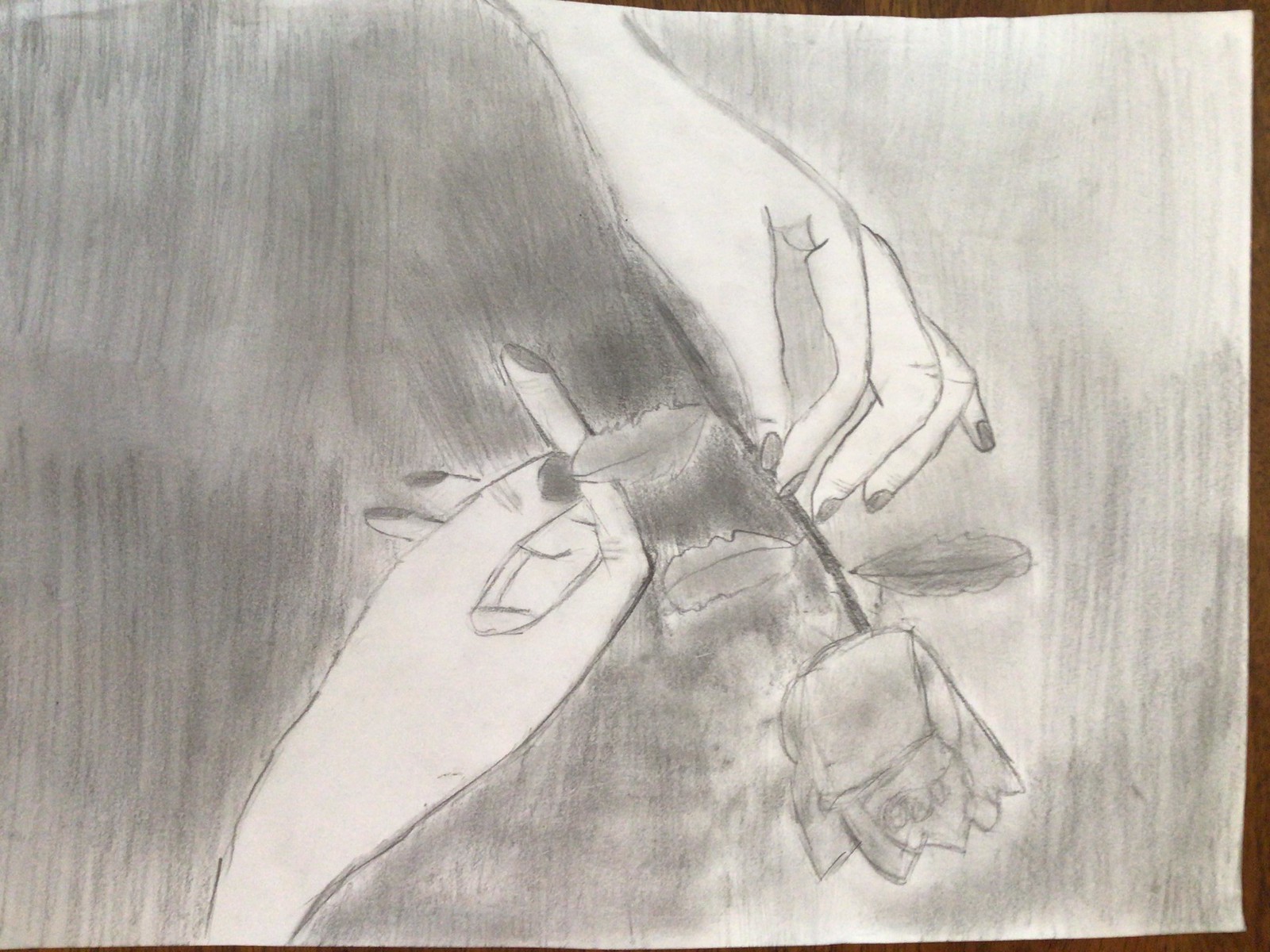This is a black-and-white sketch rendered on white paper, displayed in a photograph that has been rotated 90 degrees clockwise. The focal point is a pair of women's hands, imperfectly yet thoughtfully drawn, suggesting the work of an amateur artist or a child. The hands, adorned with visible knuckle details and nail polish, are centered as they tenderly hold a rose. The left hand emanates from the upper center of the image (which would be the left side if the photograph were correctly oriented), while the right hand enters from the lower center (the right side in the correct orientation). The rose's stem extends towards the top of the image, with the blossom facing downwards to the bottom right corner. The entire background has been densely filled in with black, likely using a thick marker or charcoal, making the delicate lines of the hands and rose stand out starkly against the dark backdrop.